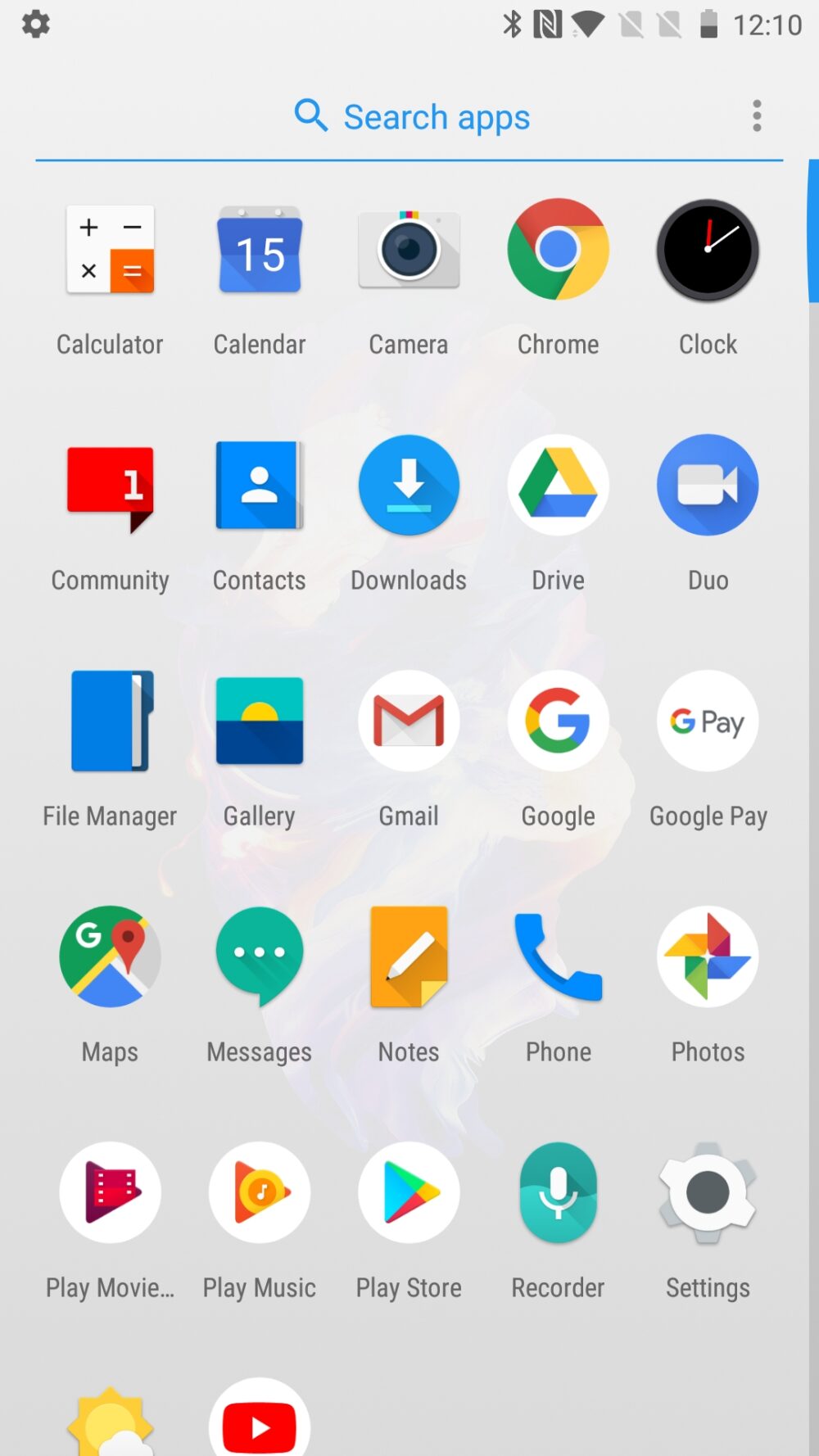The screenshot depicts an app drawer from a smartphone, capturing various details of the device's interface. At the top left corner, there is a recognizable settings gear icon. The time displayed at the top right is 12:10, and the battery icon indicates that it is approximately halfway drained. Other icons for Wi-Fi, Bluetooth, and additional notifications are also present on the status bar.

Immediately below the status bar, there is a search bar labeled "Search apps." Below this, a list of installed applications is visible. The apps displayed in the screenshot, in alphabetical order, include:
- Calculator: Icon for the calculator app.
- Calendar: Icon for the calendar app.
- Camera: Icon for the camera app.
- Google Chrome: Icon for the Chrome web browser.
- Clock: Icon for the clock app.
- Community: Possibly a messaging or social app.
- Contacts: Icon for managing contacts.
- Downloads: Icon for accessing downloaded files.
- Drive: Icon for Google Drive.
- Duo: Icon for Google Duo, a video calling app.
- File Manager: Icon for managing phone files.
- Gallery: Icon for viewing images on the phone.
- Gmail: Icon for the Gmail email service.
- Google: Icon for the Google app.
- Google Pay: Icon for the now-defunct Google Pay app.
- Maps: Icon for Google Maps.
- Messages: Icon for the messaging app.
- Notes: Icon for a note-taking app.
- Phone: Icon for the phone dialer app.
- Photos: Icon for Google Photos.
- Play Movies: Icon for the Google Play Movies store.
- Play Music: Icon for the Google Play Music app.
- Play Store: Icon for the Google Play Store.
- Recorder: Icon for the voice recorder app.
- Settings: Icon for the phone's settings menu.

Additionally, the bottom part of the list shows cut-off icons for a weather app and YouTube, whose names are partially obscured. The screenshot appears to capture a comprehensive, though not complete, view of the available apps, suggesting the person could scroll down to see the rest.